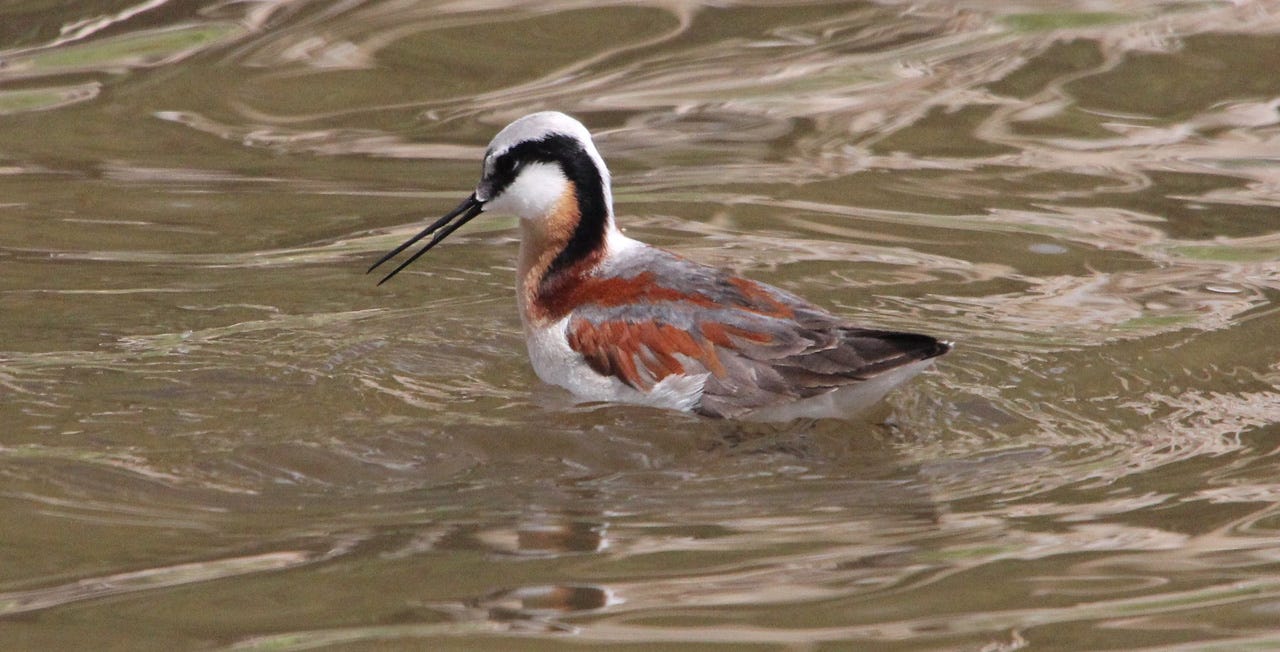This is a horizontally oriented, rectangular photograph capturing a beautiful bird, likely a swan, swimming in a body of water. The water itself is brown and appears rough, filled with small currents, eddies, and lighter white streaks topping the waves. The bird, centrally positioned and facing left, features a distinctive long, black, pointy beak with a black stripe extending back past its eye and around its head down to its neck. The bird's head is predominantly white, complementing a striking body that displays a mix of colors: reddish-brown tones on the back, gray feathers, and a white underbelly. The combination of the bird's diverse plumage and the dynamic water creates a visually captivating scene.